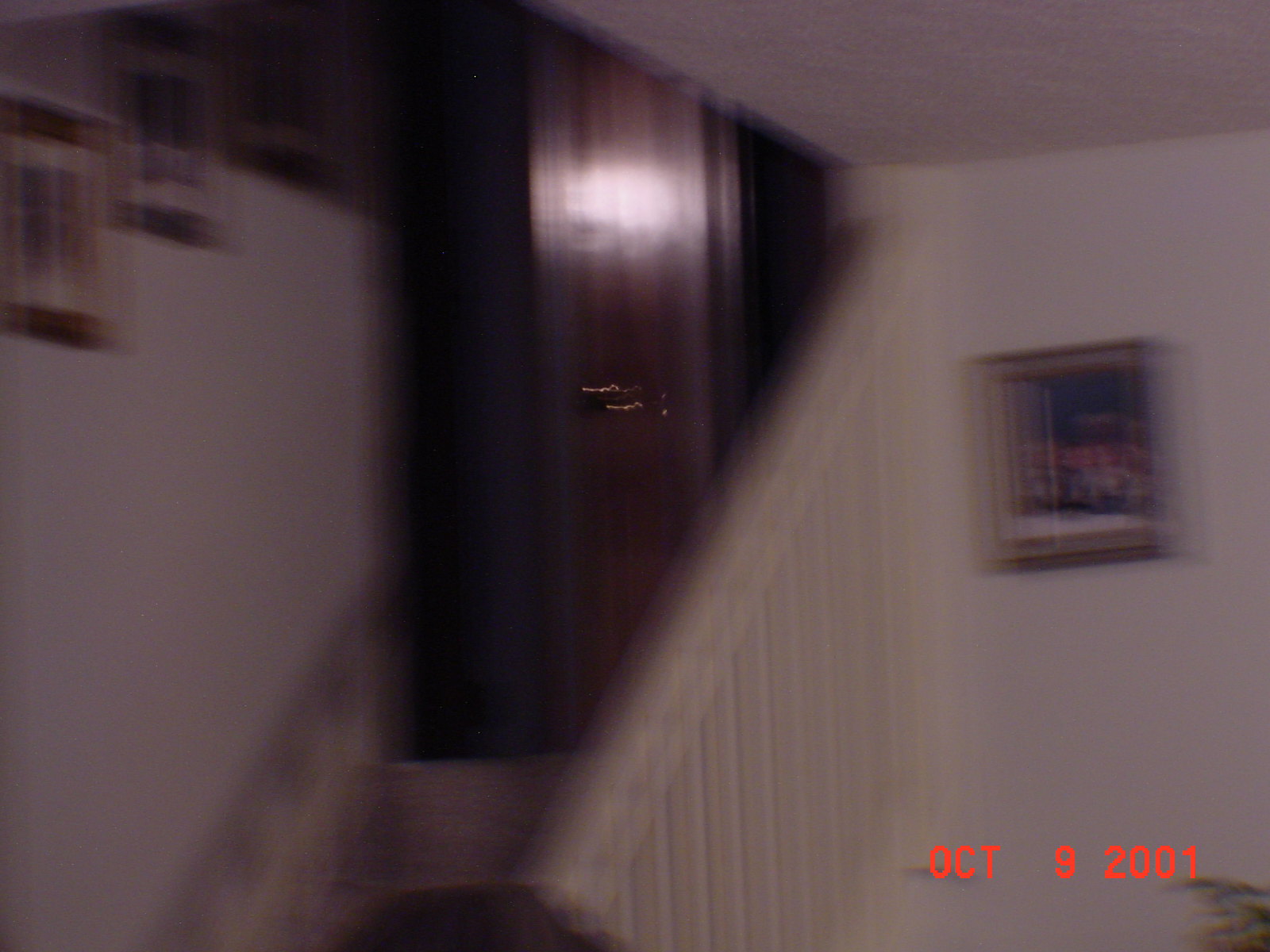This is a very blurry photograph of a small townhouse stairwell, dated October 9, 2001, in red at the bottom. The scene depicts a white-walled room with a white ceiling, featuring a white staircase banister and spindles. The stairs ascend to a top level where a brown wooden door with a gold handle is visible. Along the staircase wall, there are three framed pictures, all out of focus, and another blurry framed picture is visible on the adjacent wall when looking straight ahead. The photo's blurry nature makes it difficult to discern precise details, adding an almost ghostly quality to the scene. There also seems to be an indistinct object at the bottom, possibly the top of a person's head, barely visible and lacking facial features.